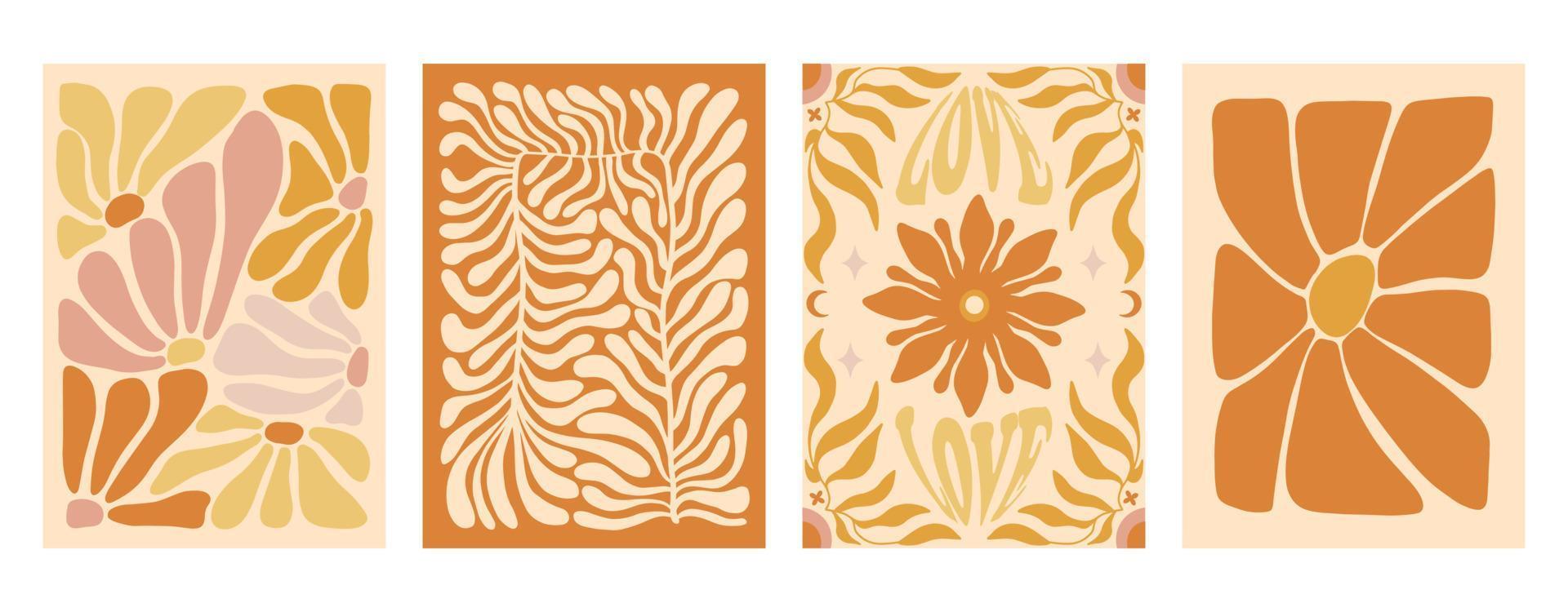The image consists of four rectangular panels arranged in a row, each resembling a wallpaper swatch with a beige background and varying patterns in shades of brown, purple, light green, subtle lavender, and creamsicle colors. 

1. The first panel on the far left features abstract flower petals in yellow, pink, shades of orange, and lavender, set against a light creamsicle orange background. The petals, depicted as halves of flowers, encompass various colors, with the middle sections ranging from orange to yellow to pink, all contained within a slight border.

2. The second panel has a deeper orange background, adorned with a design resembling a long strand of seaweed with billowy, cream-colored leaves on a stem, creating a whimsical and flowing effect. This panel also has a subtle border around its edges.

3. The third panel displays a large orange flower in the center, with the word "love" appearing above and below it, styled in a tapered fashion. The corners of this panel feature orange semicircles with small attached leaves, all blending into a light orange background.

4. The fourth panel on the far right showcases a large flower with nine orange petals and a circular yellow center. The background is a cream or creamsicle color, emphasizing the floral pattern.

Each panel contains elements of both floral and abstract designs, tied together by their similar color palettes and borders, making them suitable as coordinated wallpaper swatches.